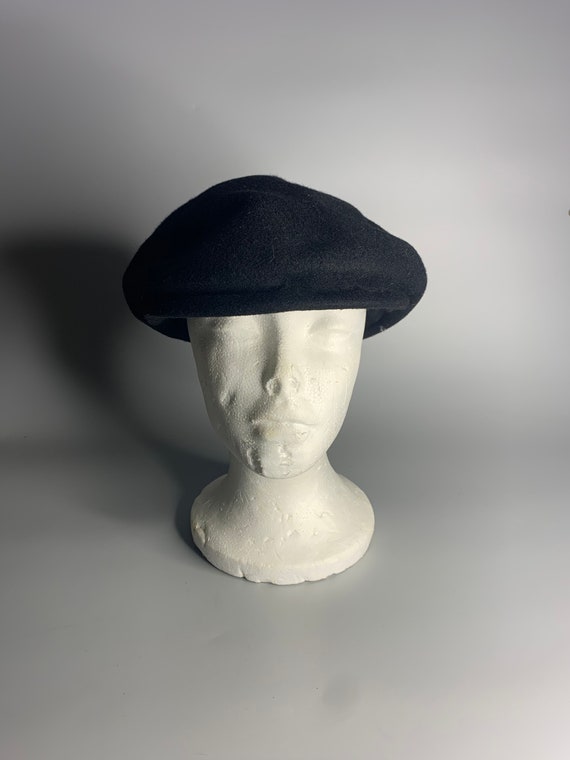The image features a professionally photographed, styrofoam mannequin head with a used, black felt hat—resembling an old-fashioned paperboy cap—perched on top. The white, androgynous mannequin, detailed with minimal facial features including indented spots for the eyes, nose, and mouth, shows wear and tear, evident from the numerous indentations, indicative of frequent use. The hat itself appears dusty and slightly dirty, with visible fibers and possibly hairs on it. The mannequin head is set against a gray backdrop, which adds a sophisticated touch to the composition, similar to an eBay product listing. The light source from the top right casts shadows to the bottom left, highlighting the texture and worn condition of both the hat and mannequin.